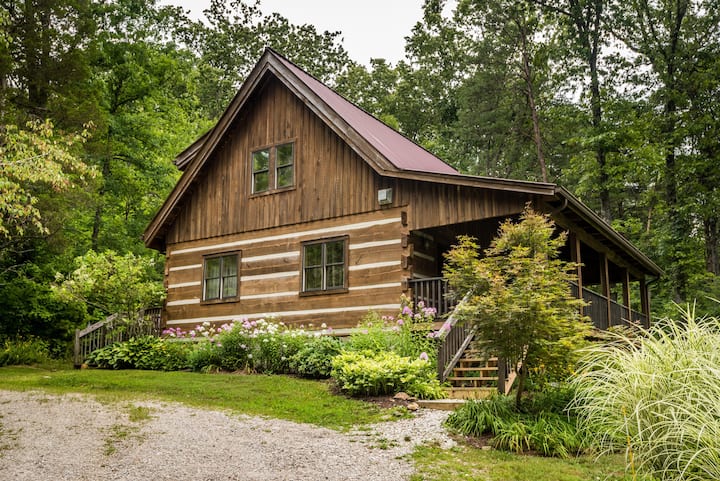This photograph captures a rustic, dark brown wooden cabin nestled in a lush forest setting. The cabin’s side view is prominently featured, with its distinctive triangular V-shaped roof suggesting a mountainous, snowy location. The cabin has a spacious, covered front porch on the right side, accessible by a set of wooden stairs. On the lower level, two four-paned windows provide a glimpse inside, while a single window is positioned centrally on the upper level. The surrounding area is rich with greenery, including tall trees, various bushes, and flowers that frame the cabin beautifully. To the left, a curved gravel driveway offers a parking area, adding to the rustic charm. The photograph is rectangular, capturing not only the detailed structure of the cabin but also the enveloping natural beauty. The background features a sky that is overcast and gloomy, further enhancing the secluded and serene atmosphere of this mountain cabin retreat.